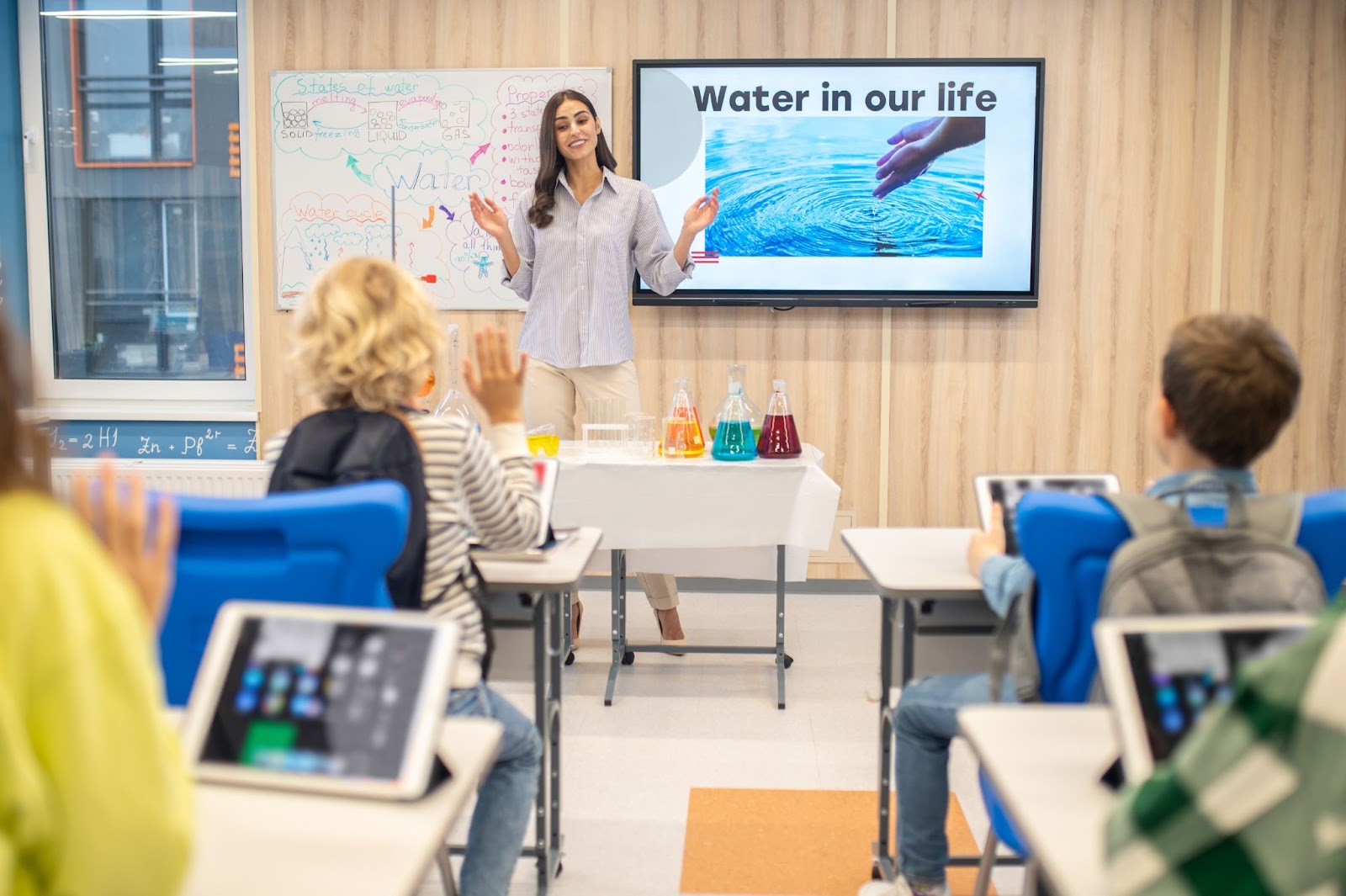The image is a clear and bright, horizontal rectangular photo capturing a classroom scene. At the front of the room, a woman, likely the teacher, stands giving a presentation. She is dressed in light-colored pants and a striped shirt. To her left is a colorful poster with a blue frame displaying an image of water with hands immersed in it, accompanied by the text "Water in Our Life." Directly in front of her is a table covered with a white tablecloth, on which various scientific containers are arranged, some filled with orange, blue, and purple liquids. A whiteboard, partially visible with marker writing, and a turned-on monitor further suggest an educational or instructional setting. On her other side, there is a partially obscured chart and a window letting in natural light. In the classroom, four students sit at individual desks or tables with their computers or tablets open, attentively facing the teacher. The room is well-lit and depicted in vivid color, contributing to the overall clarity and detail of the scene.